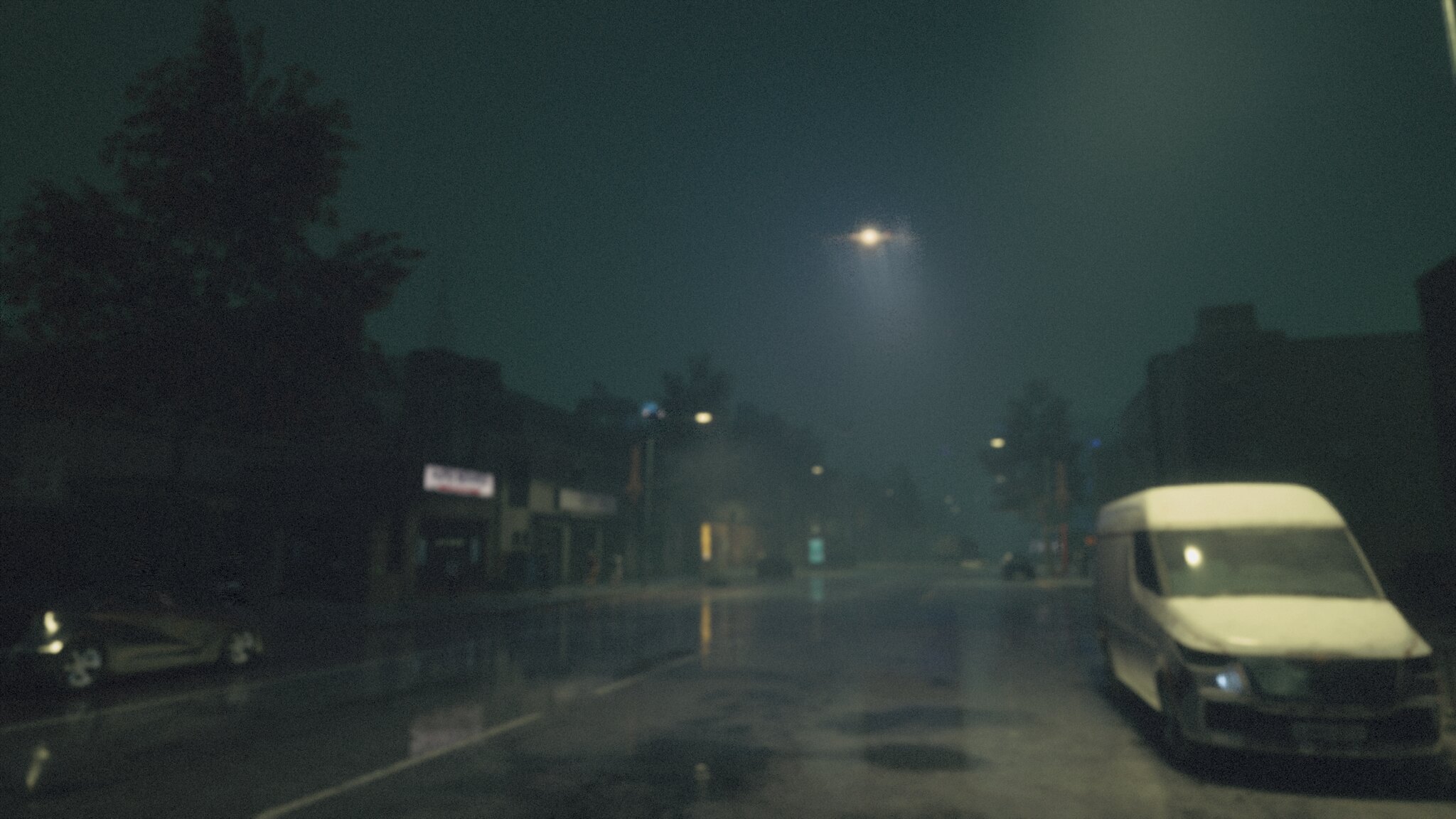This is a computer-rendered nighttime scene of a small downtown area, viewed from a straight-on perspective down the main street. The atmosphere is dim and foggy with dark, washed-out colors, indicating a recent rain that gives the street a reflective quality. On the left side of the street, there is a small sedan with its tail light glowing faintly. Further along on the right, a large white van is parked, with a round white reflection visible on its windshield. The scene features two-story buildings on both sides, likely shops, all with their lights off except for a few signs and street lights that partially illuminate the area. In the middle of the scene, floating above the street, is a solitary light source that could be a streetlight or possibly a drone. The dark sky is punctuated by the moon, shrouded in clouds, casting a subtle light over the street. Trees dot the left background and right foreground, contributing to the overall gloomy and somewhat eerie ambiance.